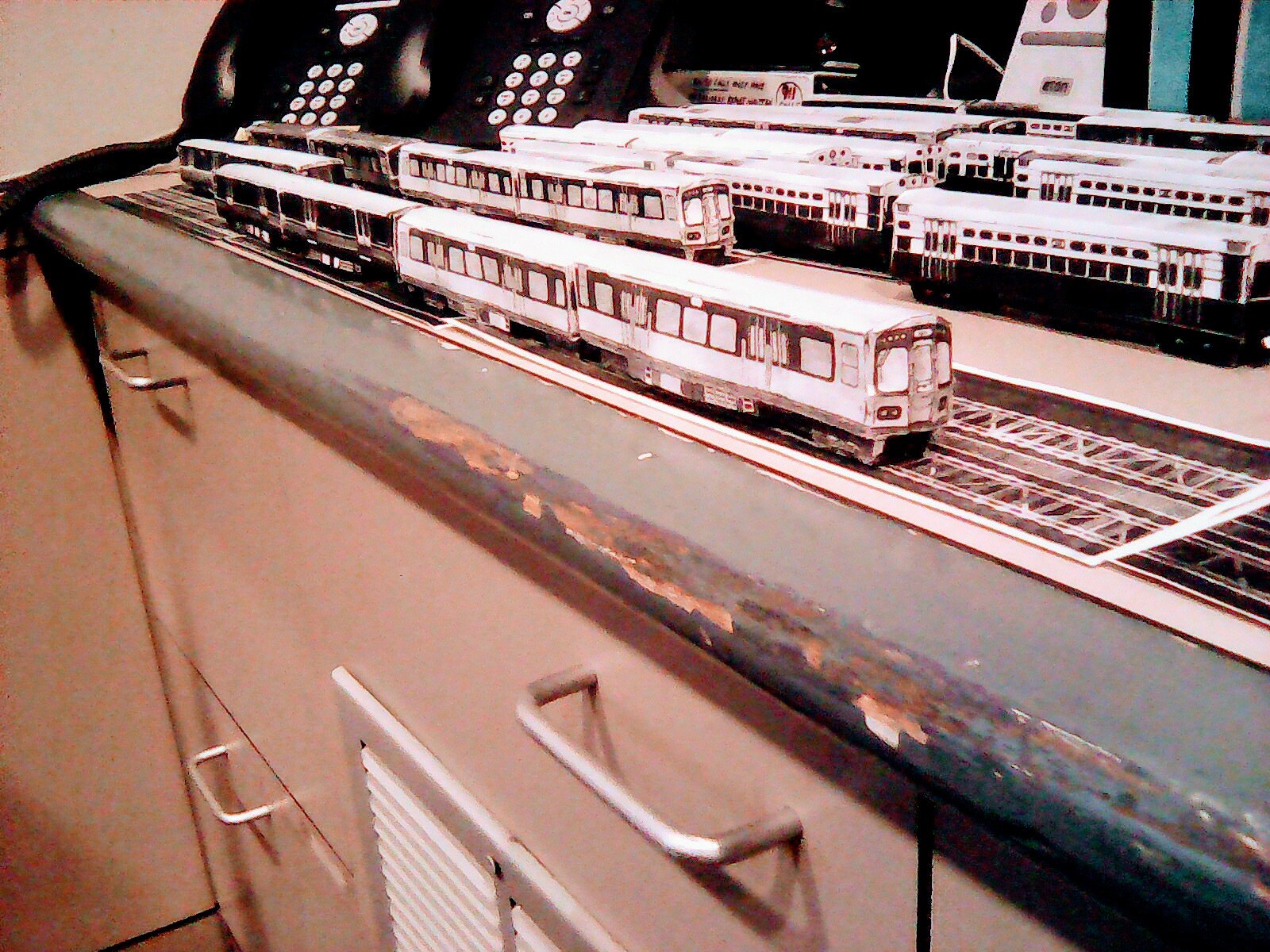The detailed photograph captures a scene on a wooden countertop, which has visibly chipped paint, situated in what appears to be an office environment. Below the countertop, there are multiple drawers and a vent, likely part of a cabinet. On top of the countertop, there are two black landline telephones with white buttons, characteristic of office use.

The main focus of the image is a set of small model trains laid out on blueprint paper spread across the countertop. These model trains, depicted in shades of black and white, give the impression of being crafted from paper and resemble detailed paper cut-outs. The models include intricate details such as black windows and some even have specific front-window designs. The trains are neatly arranged in several rows but are not placed on actual tracks.

In the background, against teal-colored walls adorned with black molding, the office setting is further evidenced. The entire scene blends the nostalgic charm of old-time toy trains with the utilitarian aesthetic of an office space.